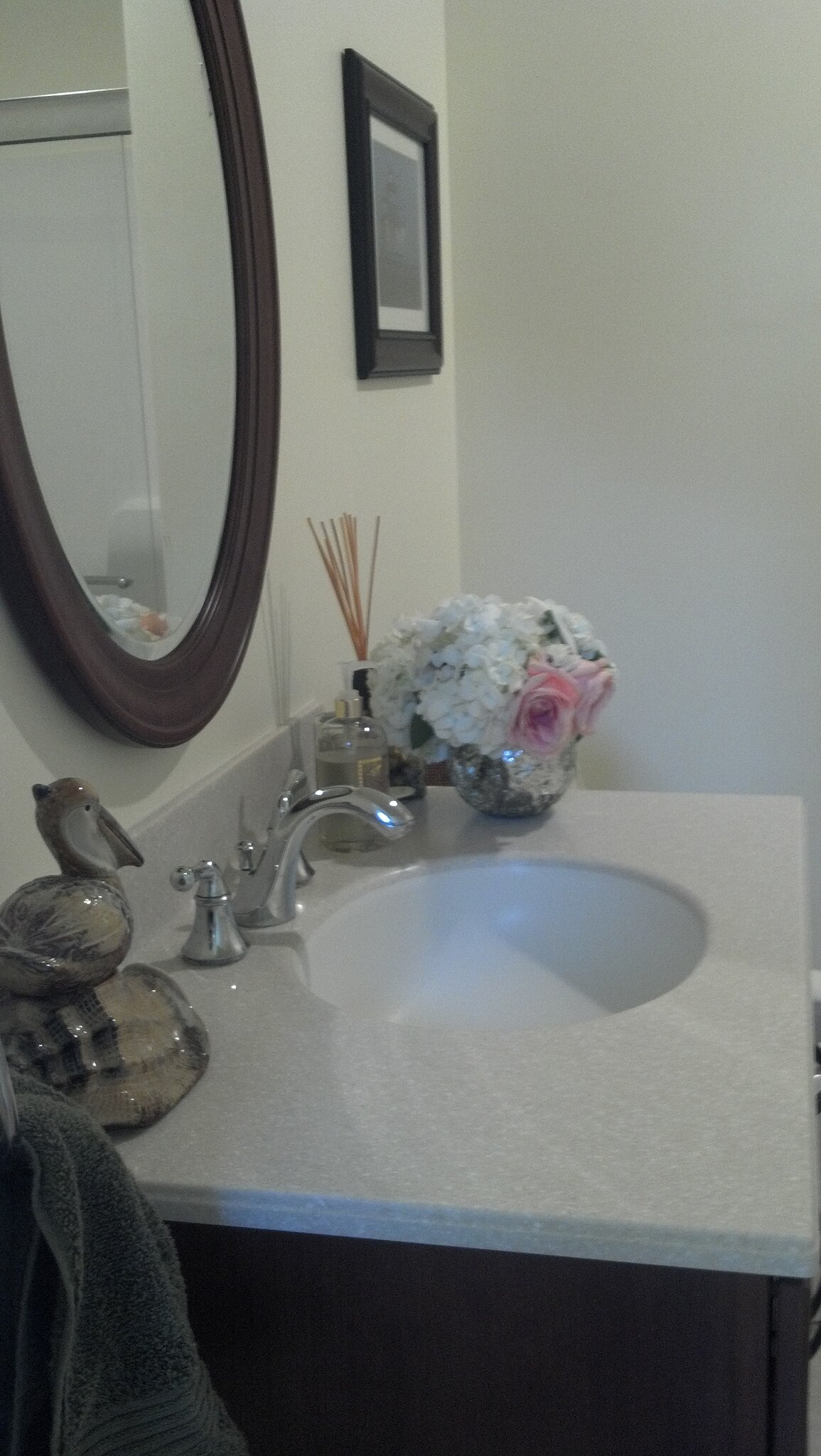The photograph captures a meticulously arranged bathroom with a marble countertop that exudes elegance. Dominating the counter is a pristine, white marble surface with a sleek chrome faucet featuring dual handles for hot and cold water. Centrally placed is a single, gleaming sink. To the right of the sink, a delicate vase overflows with vibrant flowers, adding a fresh burst of color and life. Just behind the vase, a reed diffuser subtly hints at a fragrant atmosphere. Adjacent to this setup, a hand soap pump is conveniently positioned.

On the left side of the counter, an ornate statue of a pelican perched on a log adds a whimsical touch. A neatly folded, dark gray hand towel lies next to it, complementing the neutral tones of the wood grain cabinet below. Above the sink, a vertically aligned oval mirror reflects the bathroom space, revealing a standing shower in the background. White walls frame the scene, maintaining a clean and bright ambiance. To the right of the mirror, a black-framed rectangular picture with a white trim completes the decor, adding a touch of sophistication to the tranquil bathroom setting.